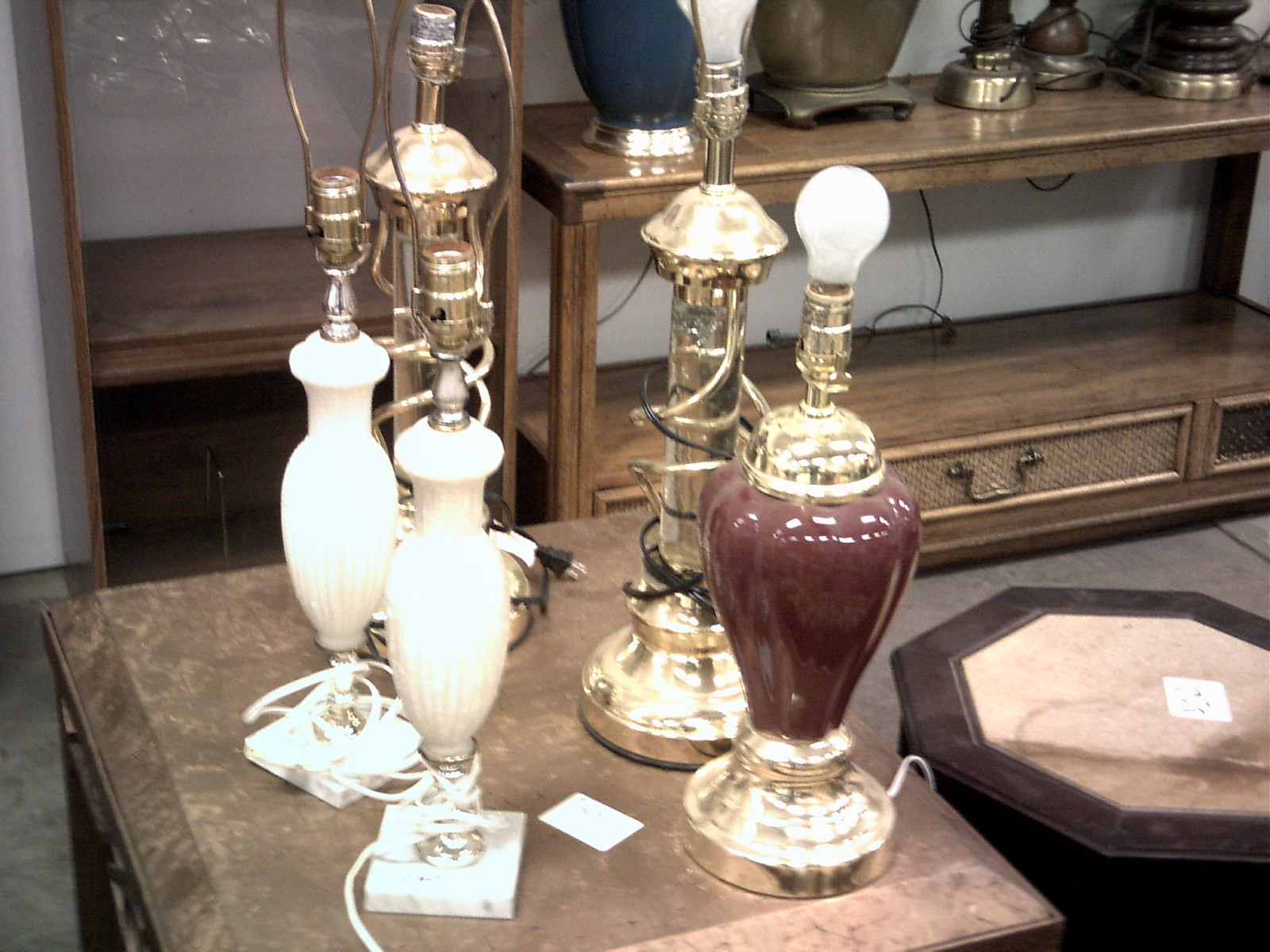The photograph, taken inside what appears to be a used furniture or antique store, showcases an eclectic collection of lamps without lampshades positioned on a brown end table with a marble-like top. Five unique lamps are prominently displayed: a red ceramic lamp with a gold base, a taller clear cut glass lamp, and two identical white lamps with spindle designs and marble bases, all with their cords wrapped around their bases. Additionally, there's mention of a marble-esque lamp which might be one of the white ones described. In the background, more lamps can be seen on a brown TV stand featuring a wicker pull drawer, though only the bottoms of these lamps are visible. Surrounding the scene is a variety of wooden furniture, including hints of a metal and wood hutch with various items piled on it, contributing to the store's cluttered and antique feel.